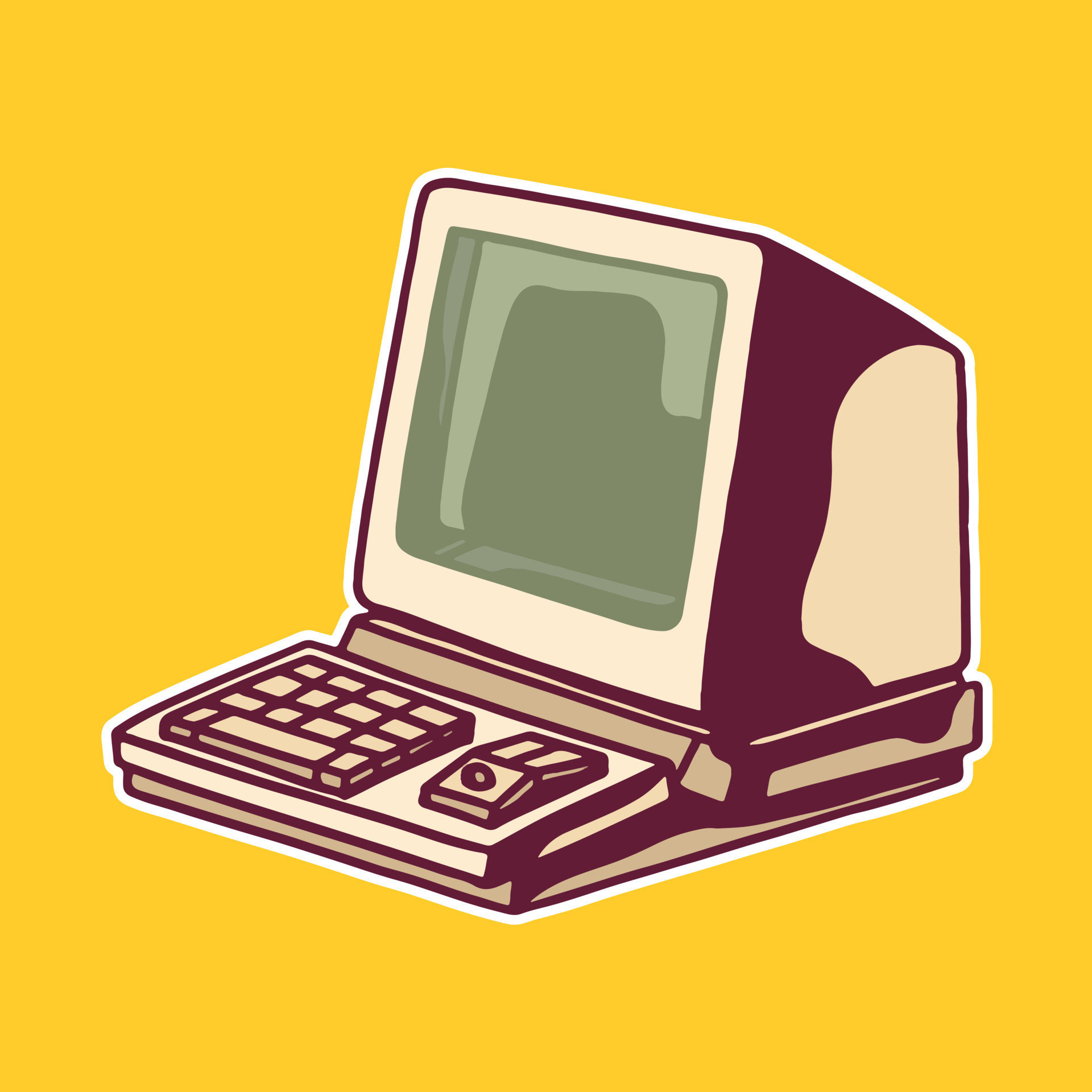The image features a detailed digital drawing of an old, clunky computer with a CRT monitor facing to the left. The entire scene is set against a bright yellow background, which adds a striking contrast to the computer's earthy tones. The computer itself is a nostalgic relic, reminiscent of vintage Mac or Commodore models. It has a green screen and an integrated keyboard, with additional buttons and keys scattered around. The monitor, together with the body of the computer, forms a single, bulky unit. A small mouse or clicker device is included in the composition, adding to the retro aesthetic. There's also a slight white border that outlines the entire image. The drawing has the rough, charming quality of a sticker or casual doodle, emphasizing the nostalgic feel of old-school technology.